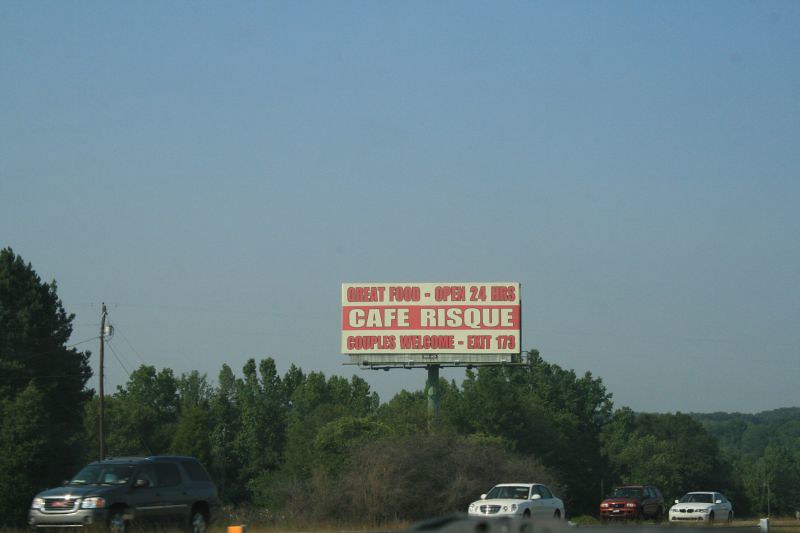The image captures a large street billboard set against an expansive sky. The sky transitions seamlessly from a darker blue at the top to a lighter blue closer to the tree line, creating a striking gradient effect. The sky occupies the upper two-thirds of the picture, while the bottom third is dominated by a dense row of trees, resembling a verdant forest. Beneath the tree line, partially obscured by foliage, is a faint hint of a road with a few cars driving along it. A gray SUV leads the line of vehicles, followed by a white car. Side-by-side behind them are another white car and a red car.

Prominently, a rectangular billboard rises on a tall pole from the trees. The billboard features the message "Great Food - Open 24 Hours" in bold red letters. Below that, within a red border and white letters, it reads "Cafe Risqué." Further down, another section with a white background and red letters announces "Couples Welcome - Exit 173." The overall scene combines elements of natural beauty with a touch of everyday life, framed by the inviting advertisement of the roadside café.